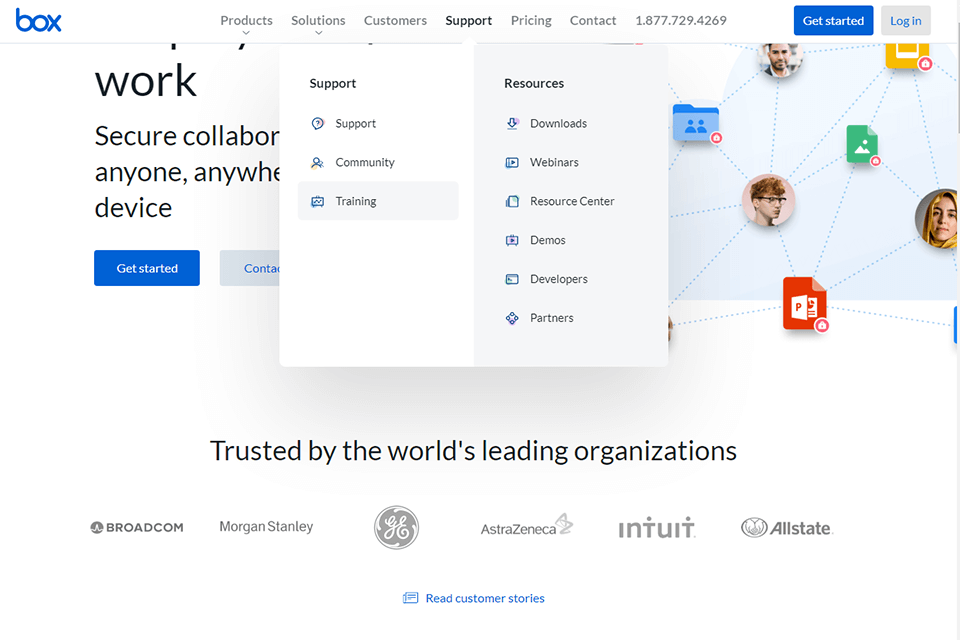The screenshot depicts a website's interface with a predominantly white background. In the top left corner, there's a blue box displaying the site’s logo or name. Adjacent to this, in gray, are expandable menu options that include "Product Solutions," "Customers," "Support," and more. These options are accompanied by a drop-down arrow indicating further navigation choices.

Highlighted are two significant action buttons: the first one is a blue rectangle with "Get Started" written in white, and beside it, a gray rectangle with "Log In" in blue text. A contact phone number, 1.877.729.4269, is also prominently displayed.

When the support tab is clicked, the screen is divided into two sections. The upper half has a white background with the word "Support" and is followed by a list of options like "Support Community," "Training," and more. The lower section has a gray background and includes "Resources," "Downloads," "Webinars," "Resource Center," "Demos," "Developers," and "Partners."

To the left, partially visible text suggests themes of work, security, and collaboration, with words like "Work," "Secure," "Collab" (short for collaboration), "Anyone, anywhere," and "Device." Below are action buttons similar to above: a blue "Get Started" button and a gray "Contact" button, though the latter is partly obscured.

At the bottom of the page, a black strip declares: "Trusted by the world's leading organizations" and lists companies like Broadcom, Morgan Stanley, GE, AstraZeneca, Intuit, and Allstate. Concluding this section, a blue text prompt says "Read Customer Stories."